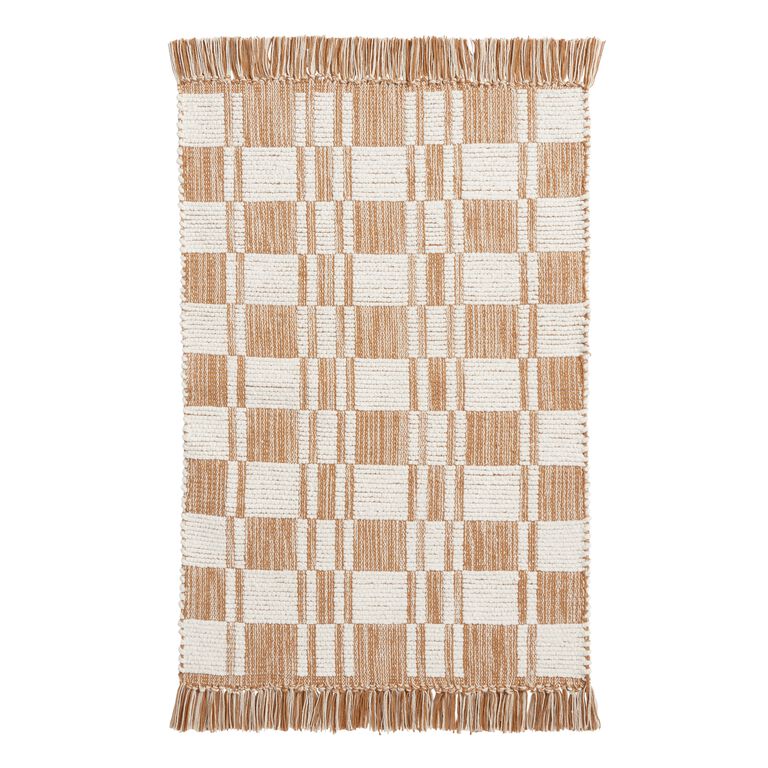This image captures a detailed photograph of a small, rectangular textile, potentially a placemat or a decorative towel. The fabric, likely natural, features a predominantly brown and white checkerboard pattern interspersed with narrow rectangular bands. Vertically oriented, the piece showcases fringed edges at the top and bottom, comprised of light brown and white tassels, giving it a finished, decorative appearance. The pattern is intricate: white squares composed of horizontal lines alternate with brown squares of vertical lines, and additional vertical brown and white striped bands intersect the main checkerboard design, creating a layered, textured effect. The left and right sides of the textile are cleanly cut, enhancing its neat, purposeful design without text or inscriptions of any kind, focusing solely on the interplay of the brown and white threads.